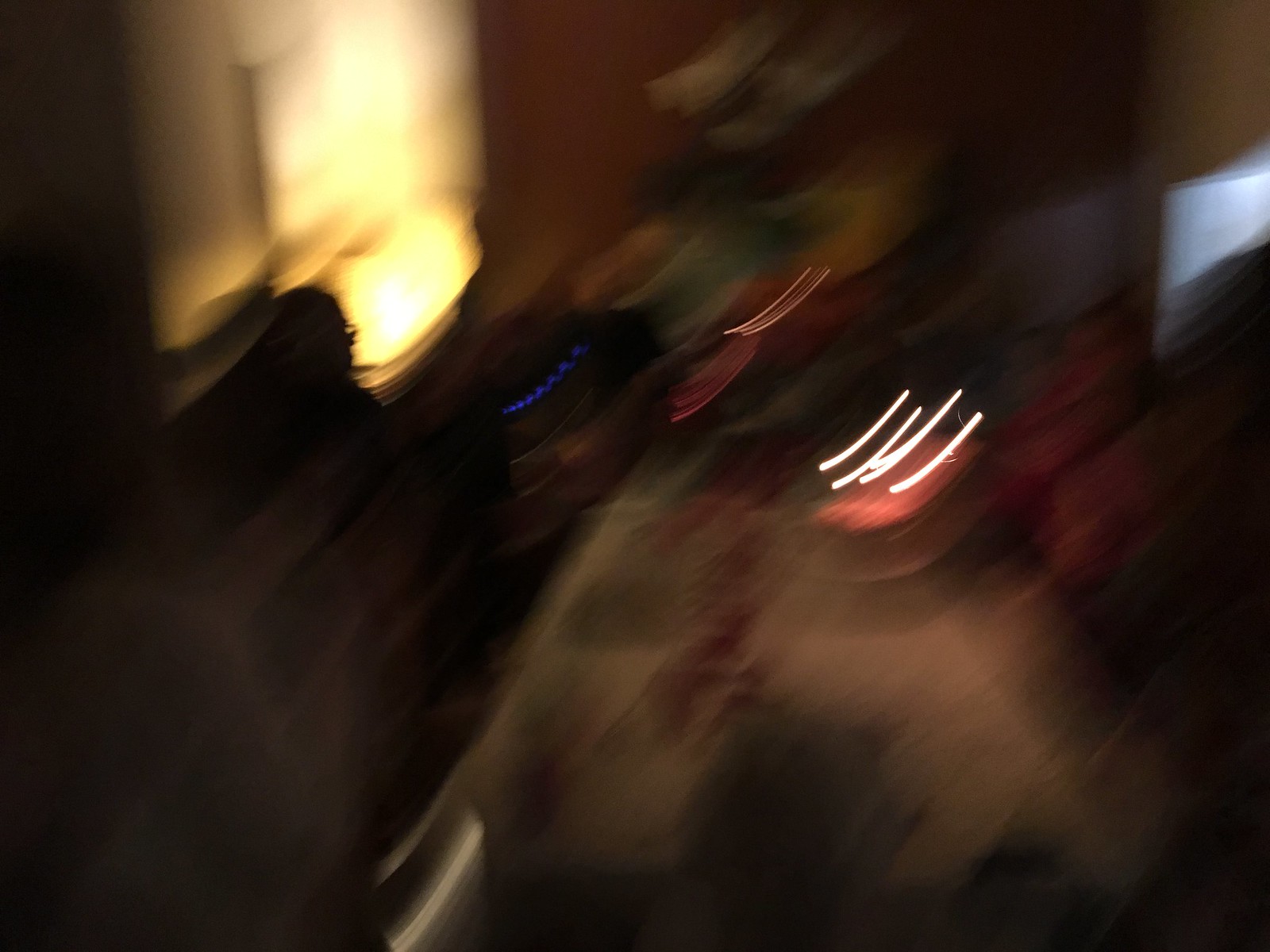A very blurry photograph captures an indistinct room where details are hard to decipher. On the left side, there is an illuminated light fixture, possibly mounted on a wall and situated atop what appears to be a wooden desk. Emerging from the left edge, a dark object, potentially the screen of a television, adds to the enigma. Near the center-right, four faint lines, seemingly the result of glare from the light, are visible. Additionally, there are small blue dots scattered towards the left-center, possibly reflections or digital artifacts.